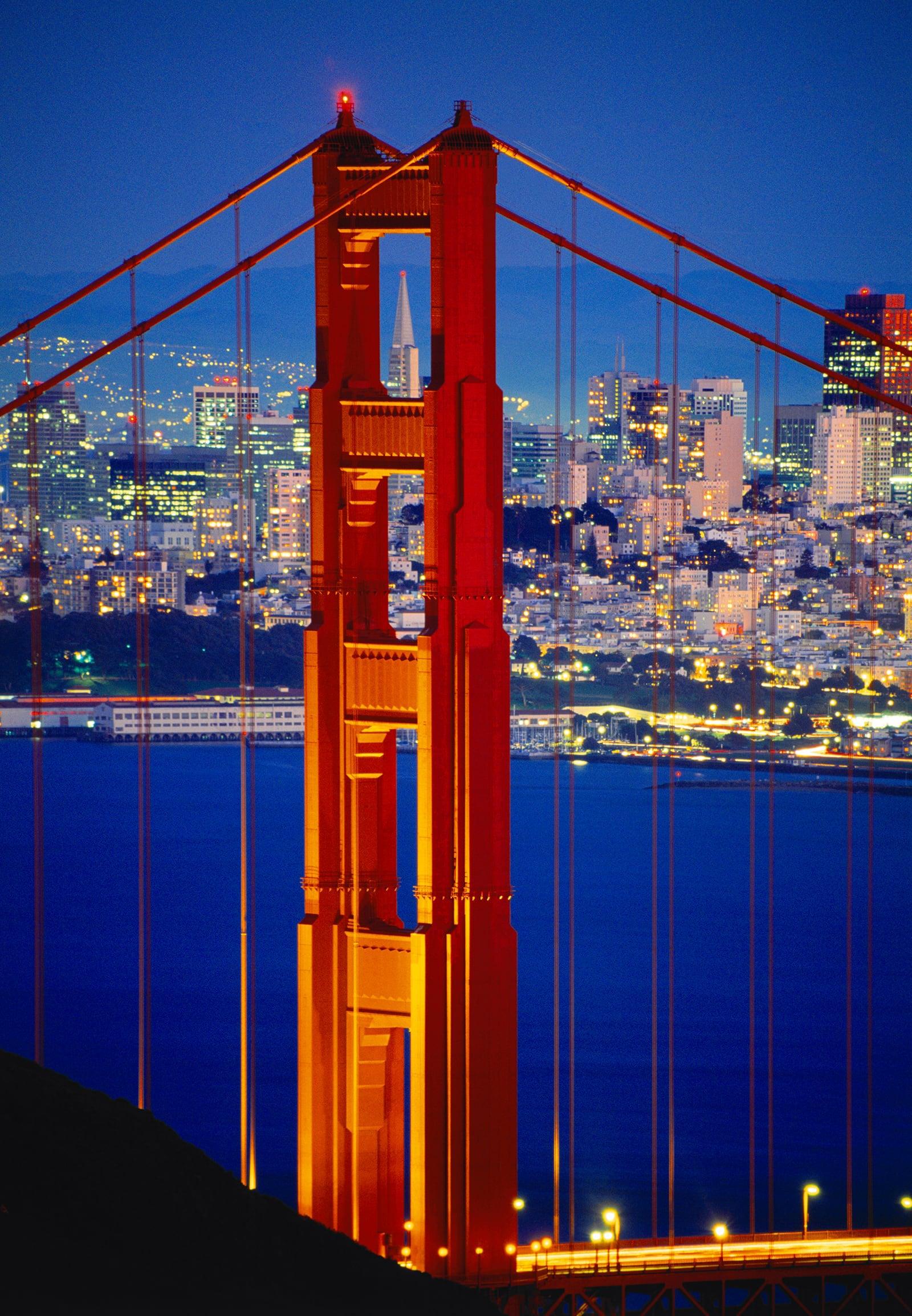This nighttime photograph captures a striking vertical view of one of the towers of the iconic reddish-orange Golden Gate Bridge, possibly in San Francisco. The dark navy blue waters of the San Francisco Bay stretch out behind the bridge, blending seamlessly with the similarly hued sky that suggests the photo was taken just after dusk. The tower, with one of its beacons illuminated red, dominates the foreground, highlighting the bridge’s cable suspension structure with its graceful cables arching up and over the tower, then radiating down to the roadway below.

The bridge itself and the streets below are illuminated with a warm orangey glow from the streetlights, casting an ethereal light on the deserted highway. In the background, a brightly lit, colorful city skyline comes into view, showcasing buildings with windows lit in shades of yellow, white, beige, and darker tones. The city lights contrast vividly against the dark blue sky and waters, and are visible from miles away, creating a vibrant yet serene urban nightscape. The photograph also features a small black section in the bottom left corner, partially obscuring the view, adding to the composition’s intriguing sense of depth and perspective. Overall, it captures a peaceful yet dynamic cityscape framed by one of the most recognizable structures in the world.